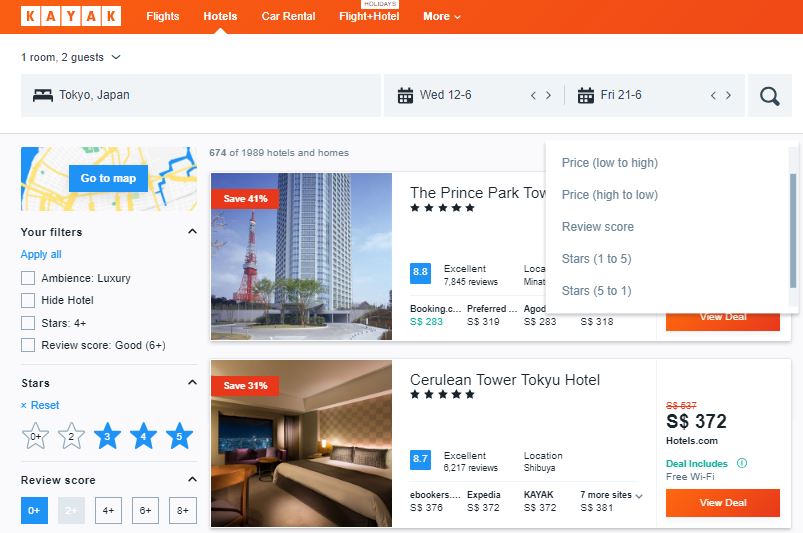This image depicts a webpage from the travel website Kayak, which is spelled K-A-Y-A-K. The interface features a distinct design with white boxes set against a vivid red background. At the very top, there's a small white box labeled "Holidays."

Beneath that, a horizontal menu includes options labeled "Flights," "Hotels," "Car Rentals," "Flight + Hotel," and a "More" category with a drop-down arrow. The "Hotels" option is selected, indicating "1 room, 2 guests." The chosen destination is Tokyo, Japan, with travel dates from Wednesday, June 12th, to Friday, June 21st.

The main section of the page displays a map, which users can access through a "Go to map" button, followed by filters that can refine the search results. These filters include criteria such as ambiance, luxury, star rating (4+ stars), and review scores (good, 6+).

A prominent section of the page shows a listing for "The Prince Park Tower" hotel, indicating a savings of 41%. A pop-up screen appears with sorting options like "Price High to Low," "Price Low to High," "Review Score," and "Stars (1 to 5)" and "Stars (5 to 1)."

Below this, details for the "Cerulean Tower Tokyo Hotel" are visible, highlighting a price of $372 available on hotels.com. This deal includes free Wi-Fi. Additional booking options are available through ebookers, Expedia, Kayak, and seven more sites, accessible via links. An orange box labeled "View Deal" allows users to explore this offer further.